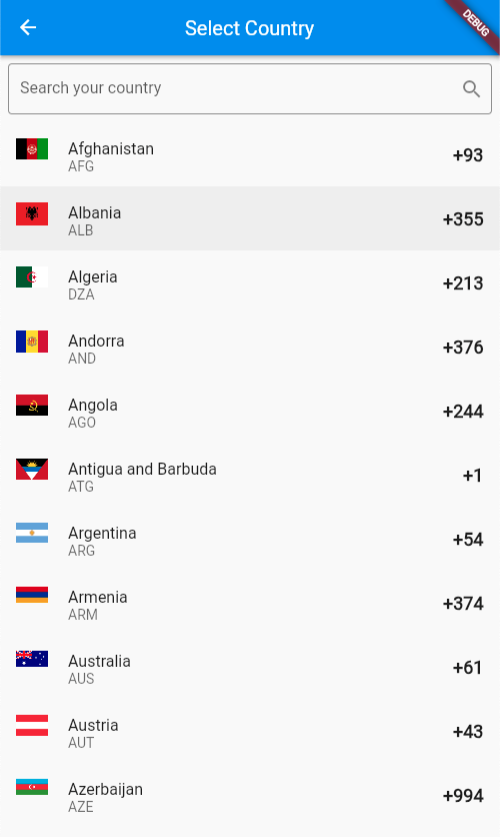This screenshot captures a user interface for selecting a country, featuring a prominent back arrow for navigation. The top section displays a brown banner labeled "debug." Below this, there is a search bar prompting users to "search for your country." The visible list includes country names and their corresponding international dialing codes: Afghanistan (+93), Albania (+355), Algeria (+213), Andorra (+376), Angola (+244), Antigua and Barbuda (+1), Argentina (+54), Armenia (+374), Australia (+61), Austria (+43), and Azerbaijan (+994). The "plus" symbol indicates the international dialing prefix for each country. The rest of the countries extend beyond the capture area and are not visible in this image.